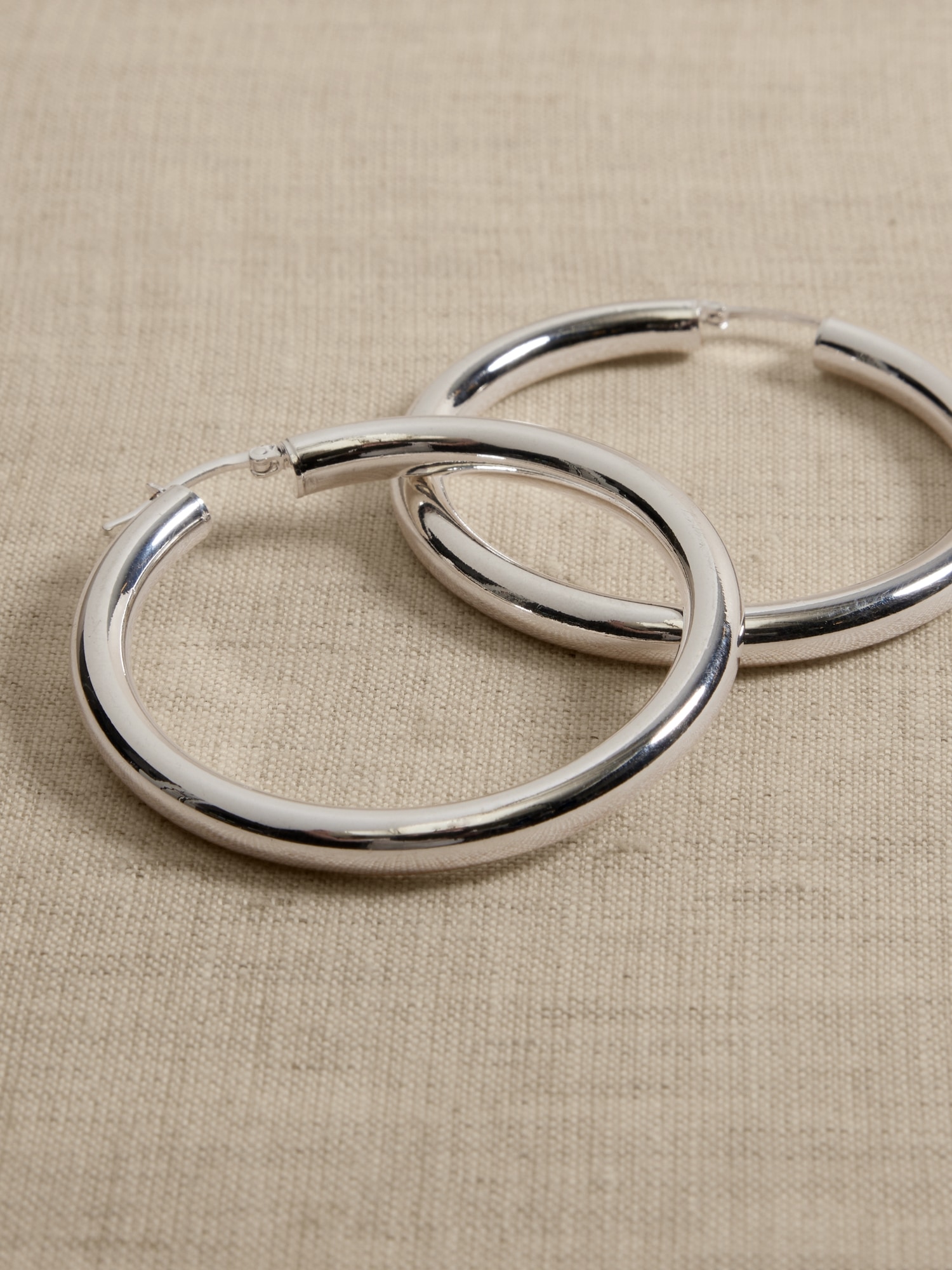This image showcases a pair of large, silver hoop earrings placed on a white linen backdrop, possibly a blanket. The hoops are arranged such that the one closest to the camera is slightly overlapping the one behind, creating an intertwined appearance. The earrings, which have a high-gloss finish, exhibit numerous reflections including some darker, shadowy elements. Each earring features a small, closed hook for securing it in the ear. Upon closer inspection, one can observe minor scratches and a slight dullness on the surface of the hoops, particularly noticeable on the bottom hoop near the point of intersection. Despite these imperfections, the earrings still maintain a generally shiny and reflective quality.